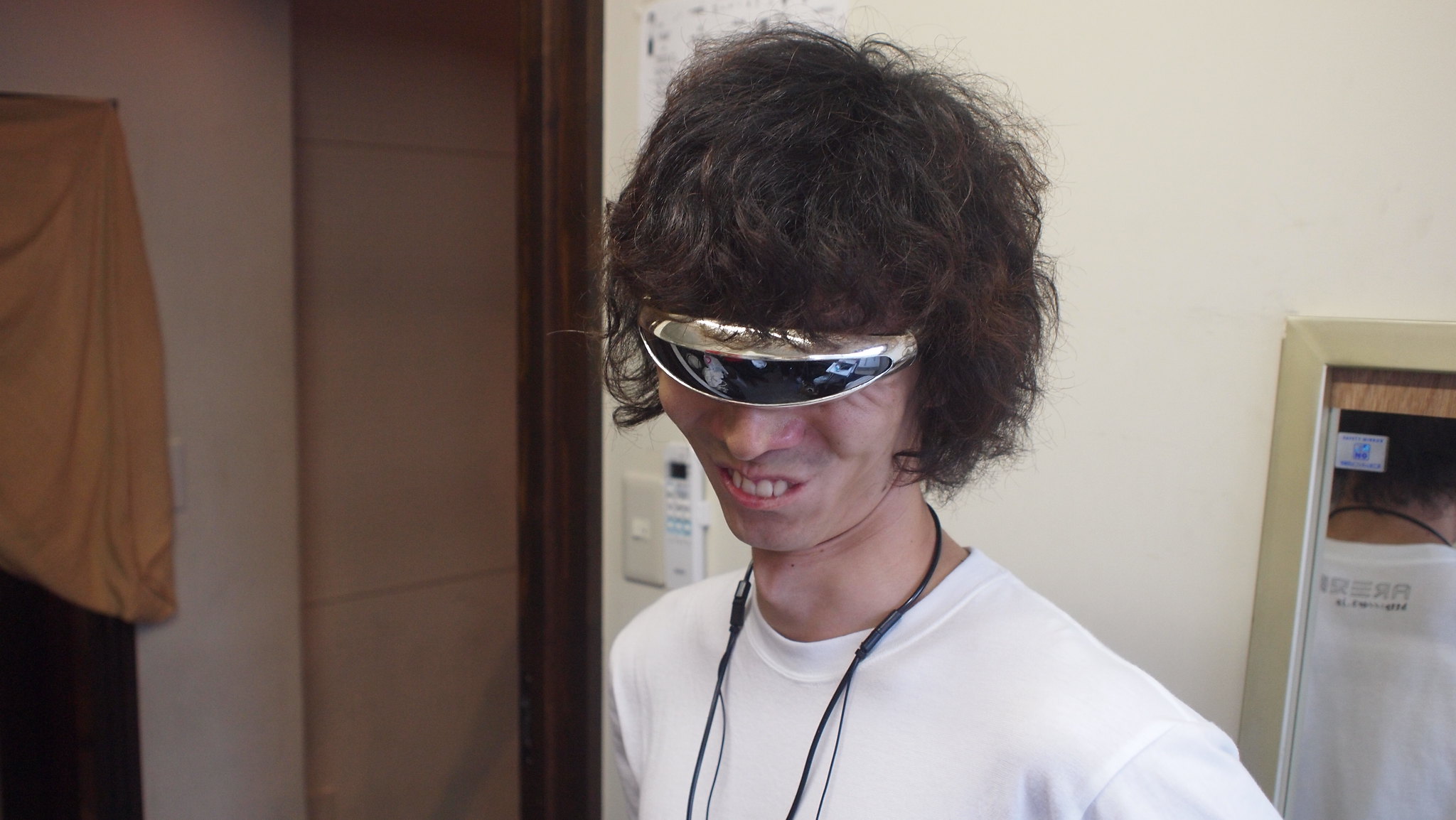This horizontally oriented color photograph captures a young man at the center, displaying his head and torso. He is wearing a white t-shirt and scraggy, neck-length, brown curly hair. His distinctive accessories include sleek, futuristic single-lens glasses with a silver rim and dark black interior, which reflect light. Around his neck, he has earphones or wires. The man sports an awkward smirk, revealing four of his top teeth, and he has a pointed nose. Behind him, a mirror reflects his back, and additional scene details include an off-white wall, a cabinet or furniture piece at the bottom right, a blurred doorway on the left, and a dark yellow blanket over furniture. Additional items in the background include a thermostat and a remote.